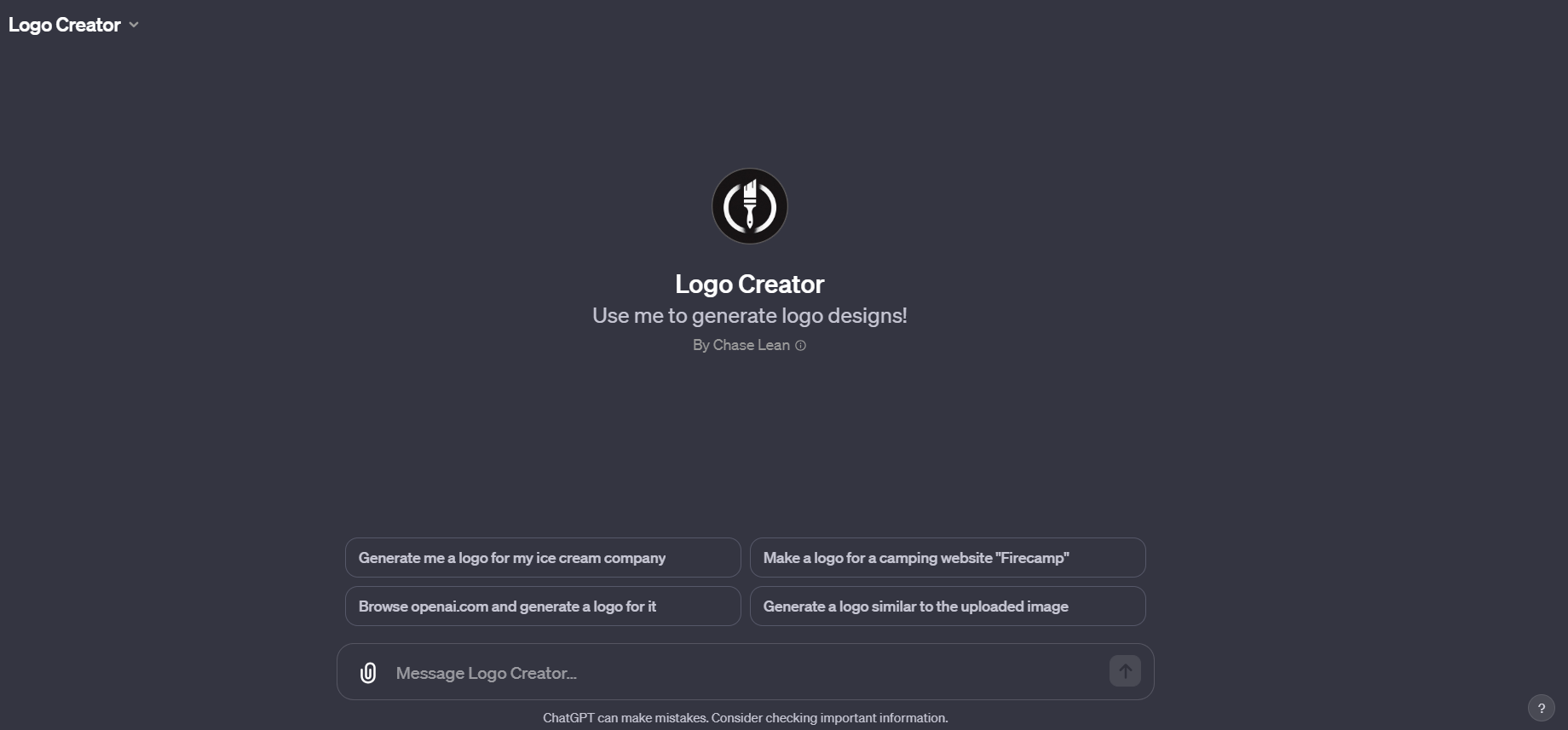The image displays a user interface for a logo creation tool branded as "Logo Creator." The background is a dark gray screen. At the center, there is a stylized icon featuring two parentheses lines framing a paintbrush and a black circle. The text "Use me to generate logo designs" is prominently displayed in white.

On the interface, there is an AI-generated text prompt area where users can describe the logo they want to create. Example prompts in white text include: "Generate me a logo for my ice cream company," "Browse OpenAI and generate a logo for it," and "Make a logo for a camping website, fire camp." Below these prompts, the interface suggests: "Generate a similar logo to upload an image."

Additional features of the interface include small, clickable boxes and a clipboard icon where users can attach logos. A message, "ChatGPT can make mistakes. Consider checking important information," serves as a reminder about the tool's limitations. On the right side, a dark gray arrow allows users to upload images. There is also a circular icon with a question mark, likely for help or additional information. On the left side of the screen, the "Logo Creator" title is displayed next to a downward-pointing arrow, which could indicate additional menu options.